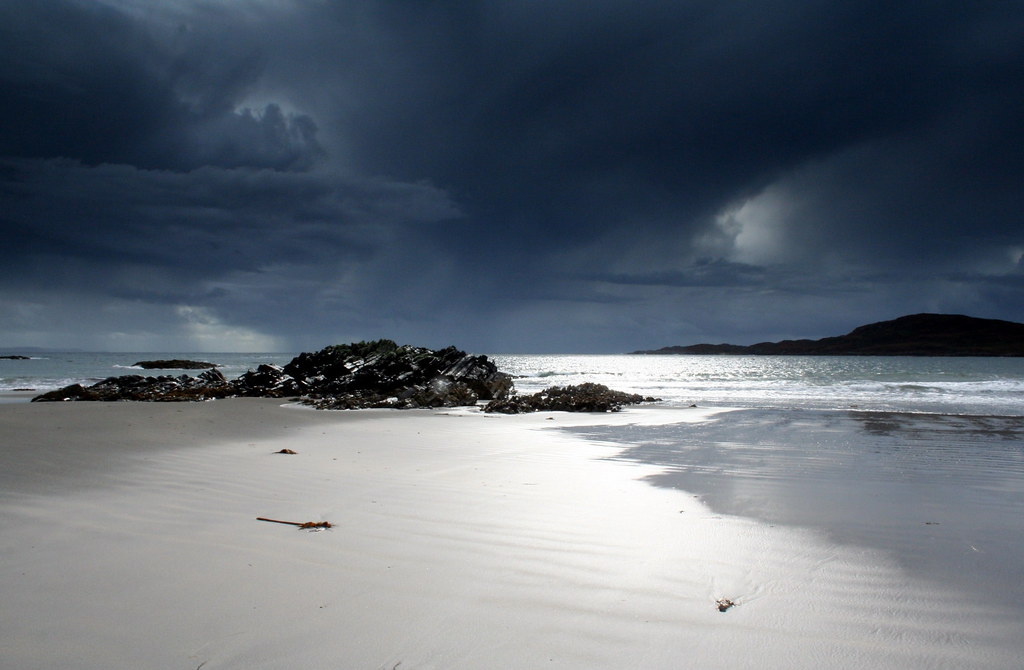This photo captures a dramatic beach scene as a storm looms on the horizon, with approximately two-thirds of the image dominated by dark, ominous clouds. Small patches of lighter sky peek through these clouds, hinting at the waning daylight. The foreground features a textured sandy beach, characterized by tidal ripples and scattered natural elements such as seaweed, black sticks, and shells or rocks. On the right side, a drainage channel adds to the intricate details of the sand. The tranquil ocean displays its reflective, light blue surface, occasionally interrupted by small waves gently crashing on the shore. Several black rocks lie at the water’s edge and further into the serene sea, indicating minimal wave activity. To the right across the water, there is a visible dark headland or possibly an island, adding to the depth of the landscape. The overall composition is rectangular, capturing the raw and untouched beauty of the coastal environment under the threat of an impending storm.